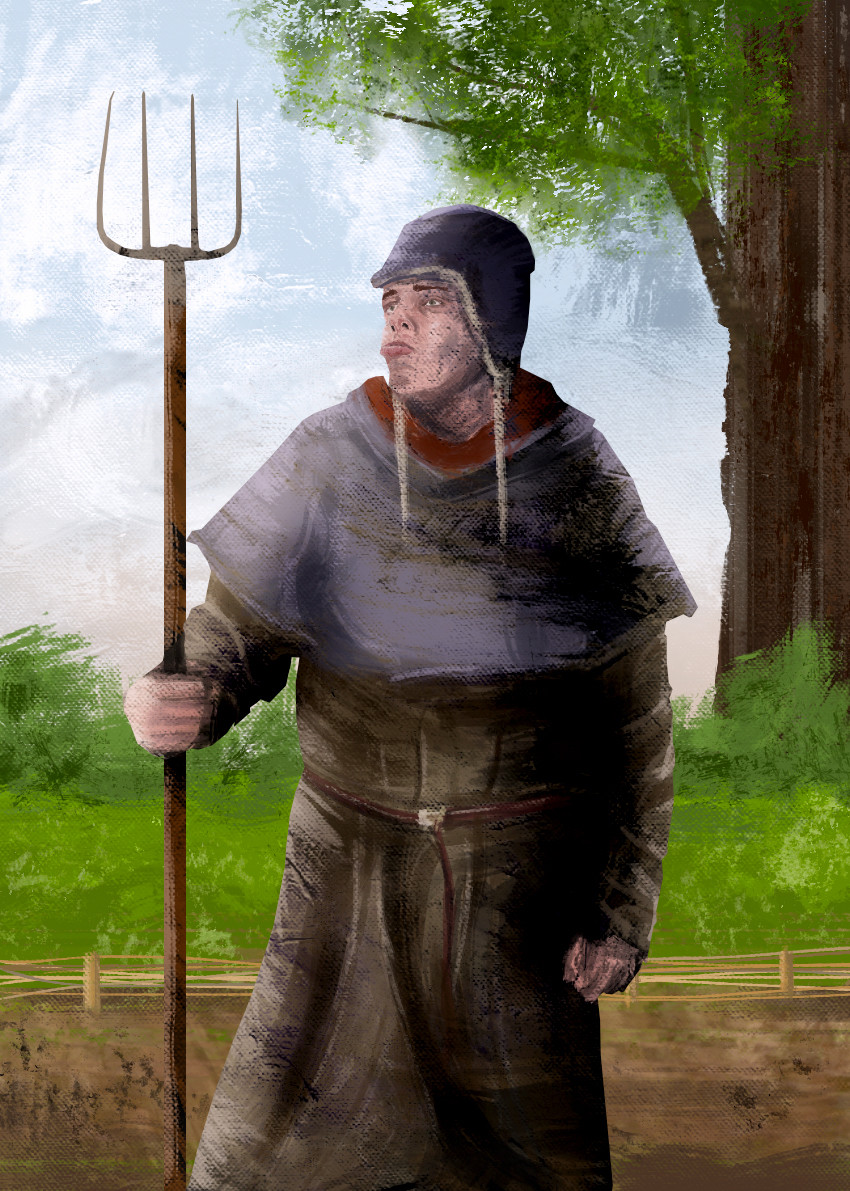The image portrays a detailed painting of a medieval man at the center, holding a large pitchfork in his right hand. The man appears to be a Caucasian peasant, clad in a brownish robe belted at the waist, and draped with a bluish-purplish shawl. He also wears a matching bluish-purplish hat with two hanging braids or strings. His expression shows a puckered mouth as he gazes toward the top left of the painting. The pitchfork, slightly taller than the man, features four prongs. The background is a rural landscape with vibrant green grass, a small fence, a large tree on the right, an overcast sky, and dirt beneath his feet, planting the scene firmly in an outdoor setting.